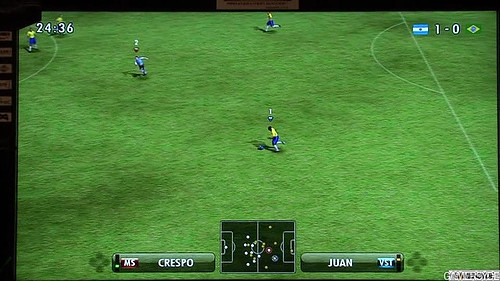The image captures an intense moment in an ongoing soccer video game. The scene features two teams, one decked in white jerseys and the other in yellow. Prominently displayed on the left of the screen is the name "Crespo," while "Juan" is visible on the right, indicating the players involved. The scoreboard in the upper right corner shows a tight match with a score of 1-0, and the game clock reads 24 minutes and 36 seconds. The players are actively engaged on a vibrant green field, with one athlete in a yellow jersey taking a pivotal action. This player, poised mid-motion, has one foot pulled back, ready to propel the ball forward, with his shadow perfectly cast on the lush grass and over the ball, adding a realistic touch to the scene.